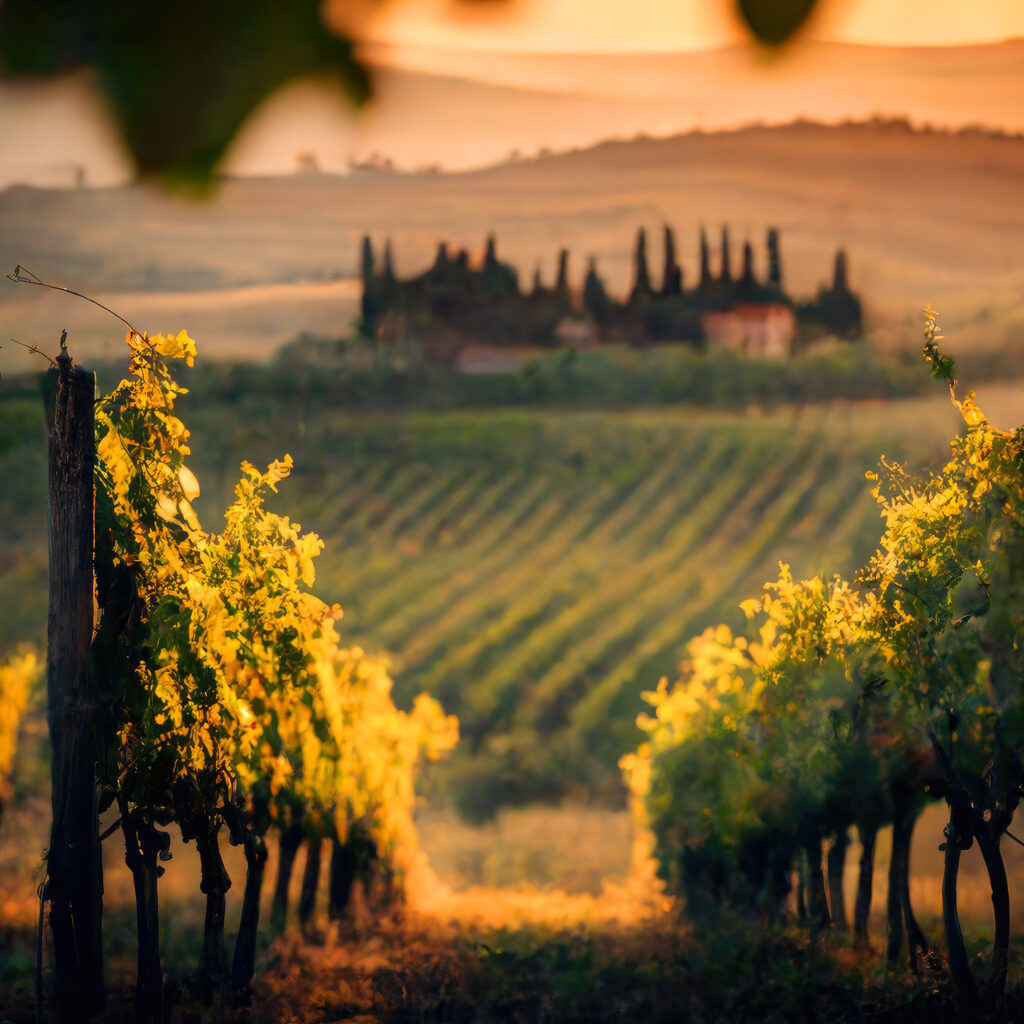The image captures a picturesque vineyard bathed in the golden light of either sunrise or sunset, giving the scene a warm, yellowish tint. In the foreground, rows of grapevines, supported by wooden posts, stretch out on both the left and right sides, leading towards a central clearing that allows for passage through the crops. The lush green vines demonstrate vibrant growth, indicating a healthy vineyard maintained meticulously for wine production. As the rows of grapevines extend into the distance, they merge seamlessly with a vast field and eventually give way to a series of rolling hills and a distant mountain range, shrouded in a peachish hue from the low sun. In the middle ground, partially obscured by the blur of distance, there are white buildings with reddish-brown roofs, possibly serving as wineries or related facilities, silhouetted by dark, towering trees behind them. The entire scene is framed by a few leaves at the top of the image, casting shadows and adding a touch of depth to this serene agricultural landscape.